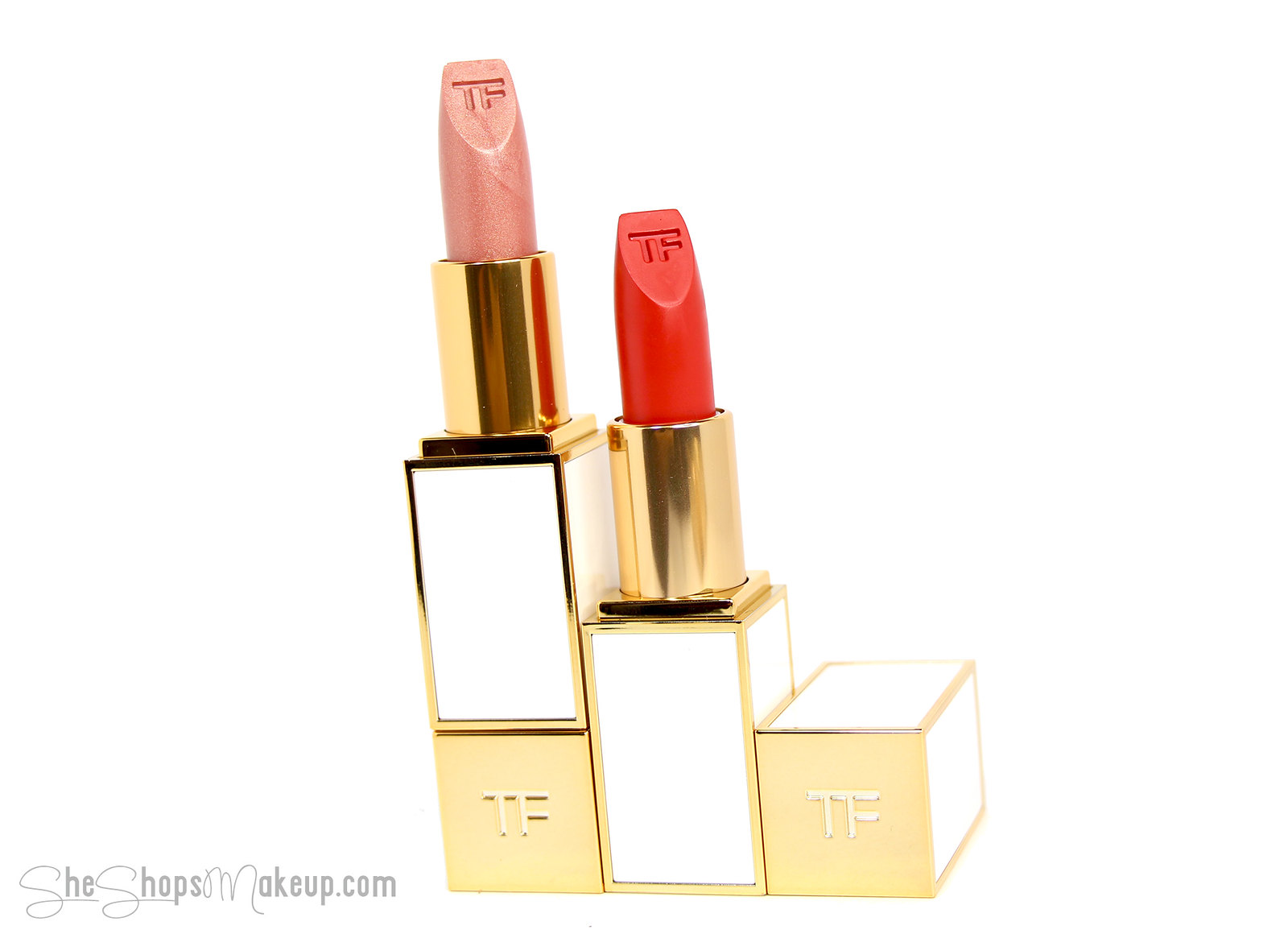The image showcases a tiered arrangement of luxurious lipsticks against a clean white background, resembling a staircase ascending from right to left. At the bottom left, the text "SheShopsMakeup.com" is prominently displayed. Each tier features a beautifully designed box and lipstick combination.

On the lowest tier, a small white box trimmed in gold, with "TF" inscribed in the pink section, sits elegantly. Next to it on the next tier up, there is a shorter white and gold box housing a classic red lipstick, extended to showcase its full length, with "TF" imprinted on the case. The highest tier features a larger white box with gold trim and a pink frosty lipstick extending from its gold-accented tube, also marked with the "TF" insignia.

The arrangement of the lipsticks echoes a stair-step pattern starting from the smallest box on the right and ascending to the largest box on the left, providing a sophisticated display of the makeup products.